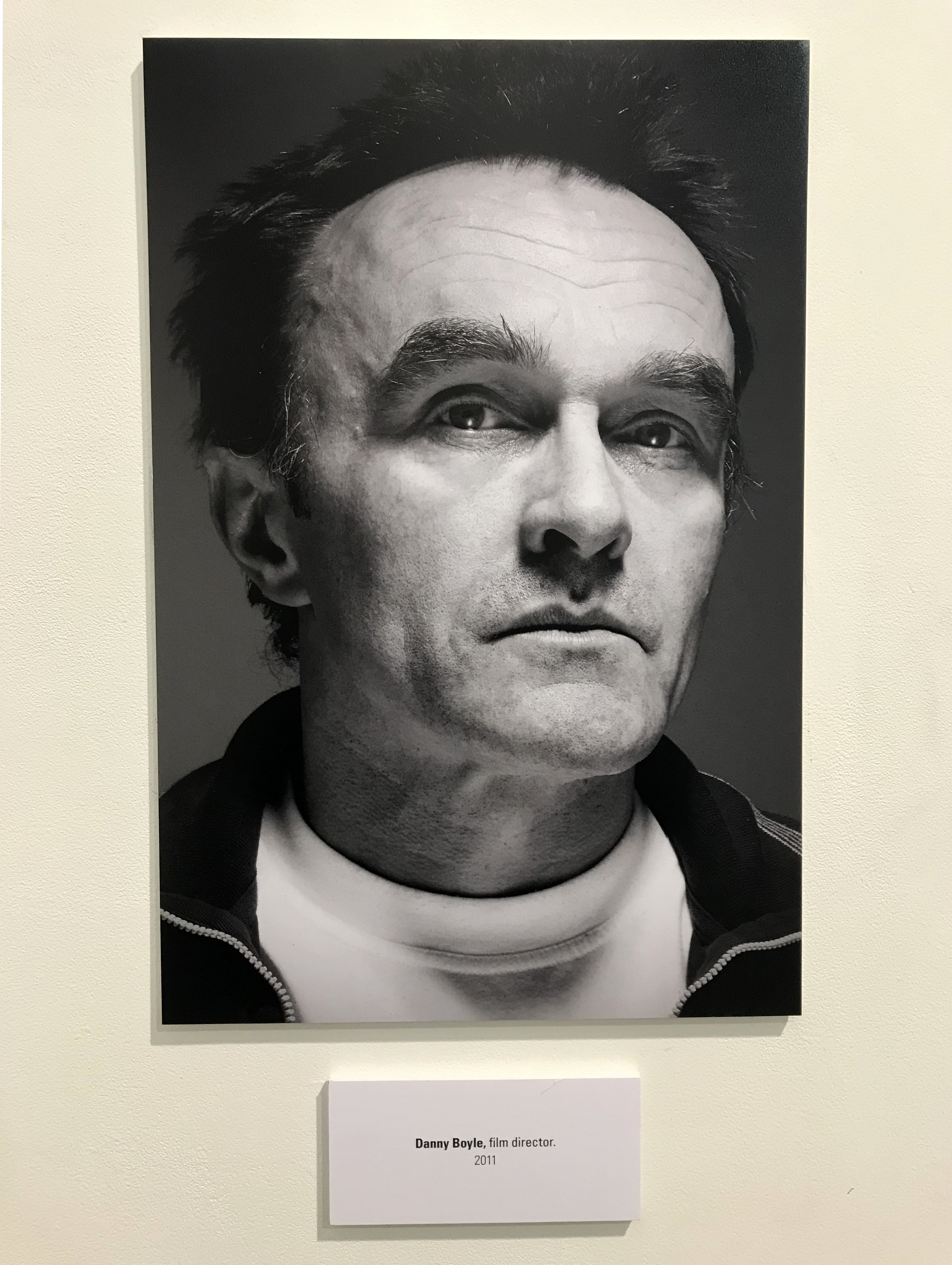The image is a horizontally aligned photograph depicting a black-and-white portrait of an older Caucasian man, possibly a film director, with a sharp focus on his facial features. The photograph is centered within a light gray rectangular background that extends beyond the image, creating a sense of depth with a slight drop shadow along the bottom and left side. The man, who might be in his early 50s or 60s, has a distinctive appearance with heavy forehead lines and a receding hairline, his combed back or blown back dark hair forming a slight spiky pompadour. He is dressed in a black collared jacket with a white lined zipper or stripe detail over a high-necked white shirt. His head is turned towards the viewer’s right, revealing the left side of his ear but obscuring the right. The character lines on his face imply he's looking off into the distance. Underneath the photograph, there is a horizontally aligned, three-dimensional appearing placard in a light gray color with a white border at the top and darker gray borders on the left and bottom. The placard features bold black text that reads "Danny Boyle, film director," followed by finer print possibly denoting years such as "2011" or "2013." This meticulous detail and modern style suggest the photograph could have been taken within the last 25 years, despite being rendered in black and white.